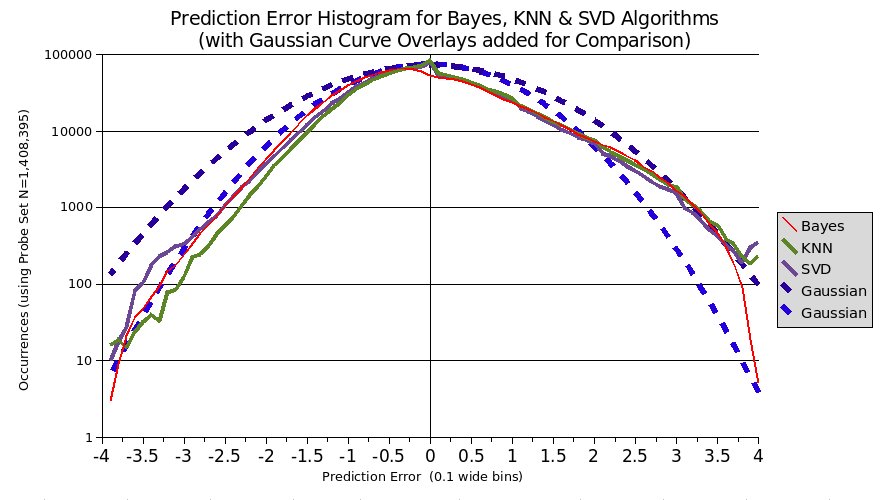The image depicts a detailed prediction error histogram comparing the performance of Bayes, KNN (k-nearest neighbors), and SVD (singular value decomposition) algorithms, with Gaussian curve overlays added for comparison. The x-axis illustrates prediction error, segmented into 0.1 wide bins ranging from -4 to 4, while the y-axis represents occurrences, using a probe set size of 1,408 for weight and 1,408,395 for set. The graph features a white background and a grid layout of two columns by five rows, labeled up to 100,000 occurrences. Each algorithm is color-coded: red for Bayes, green for KNN, and blue for SVD, with the Gaussian curves displayed as slightly darker and smaller dashed lines. The curves of each algorithm and Gaussian overlay create a rainbow-like pattern, peaking around 100,000 occurrences, indicating the frequency distribution of prediction errors from the negative to positive spectrum.